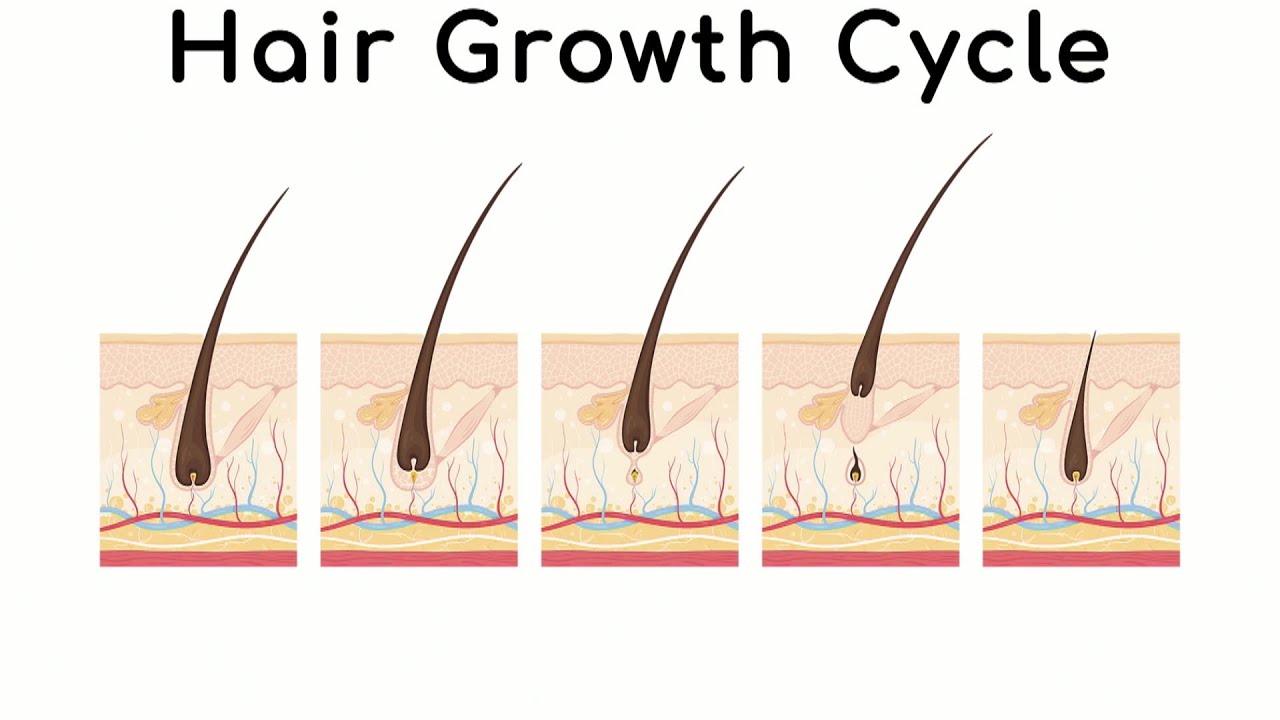The image appears to be an excerpt from a medical textbook, likely focused on dermatology, detailing the hair growth cycle. Across the top, the caption "Hair Growth Cycle" is prominently displayed. The sequence consists of five illustrations from left to right, depicting various stages of hair growth and shedding.

- **Image 1**: This initial illustration shows a fully formed hair strand intact and embedded within the skin.
- **Image 2**: Here, the hair appears to be at the beginning stages of shedding, slightly elevated from its initial position.
- **Image 3**: The third image continues to illustrate the hair as it further recedes and thins, moving closer to the skin's surface.
- **Image 4**: In this stage, the hair looks to be nearly expelled from the skin, indicating it is almost entirely shed.
- **Image 5**: Finally, the last image depicts a new hair follicle beginning to emerge, suggesting the cycle is restarting with a new hair growing while the old one has been pushed out.

Overall, the series of images provides a detailed visualization of the hair growth and shedding process, highlighting the continuous renewal cycle of hair.